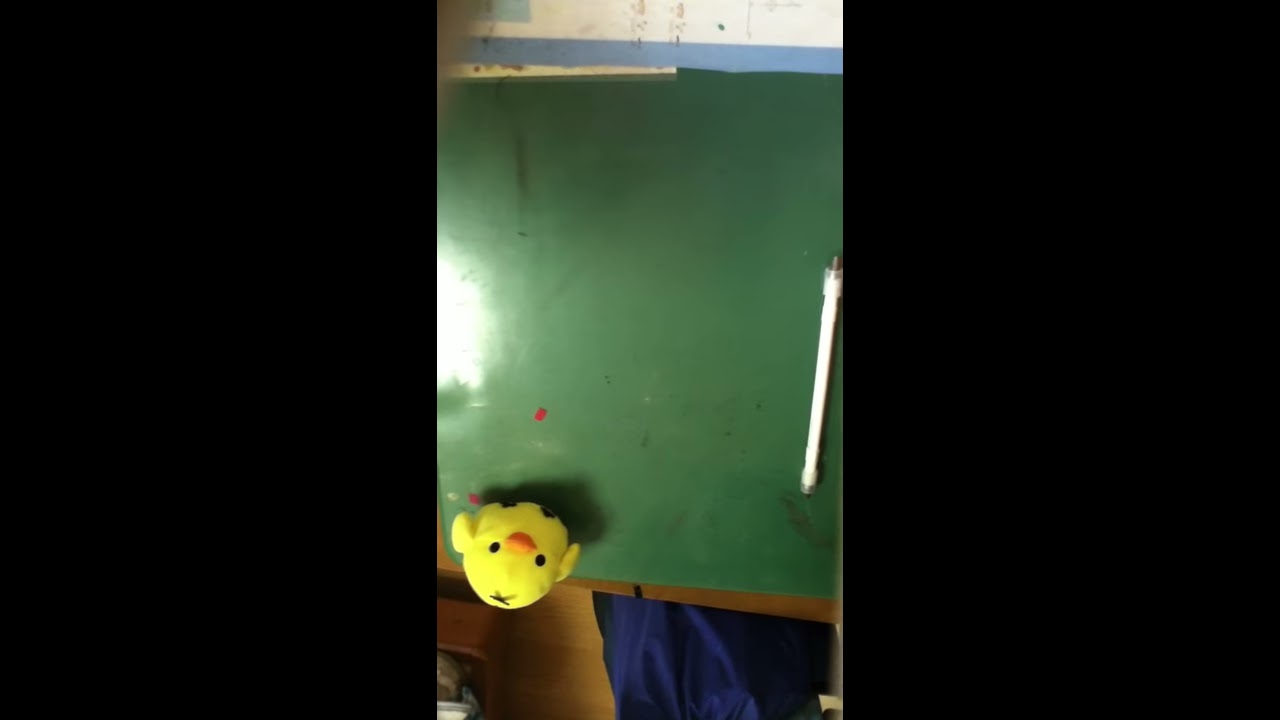This is a horizontally rectangular image, potentially a screenshot from a video or security camera footage taken indoors. The main focus is a central smaller rectangle surrounded by very wide black bands on either side, with some lights near the black borders. The background of this central rectangle is predominantly green, which might be a green tablecloth on a table.

In the lower left-hand corner of this rectangle, there's a small cartoon-like person with a green face and black hair sticking up in all directions. This character has visible ears, eyes, and a mouth, with a distinct red area in the center of its forehead. The figure appears to be wearing something brown, and there's a curving shape in the background behind it.

Towards the right-hand side of the image, there is a white pen lying on the green surface. Also present is a yellow plush duck or chick, with an orange beak and two black eyes, sitting atop the same surface. Near the bottom of the image, something blue is sticking out. 

The image further shows that beneath the green surface, there is cardboard or paper in white and blue colors visible, adding to the complexity of the details captured. Additionally, the photographer can be seen wearing blue jeans, and the image partially reveals a wooden floor. The upper part includes a blue line and some white areas, which are not very clear but add ambiguity to the overall scene.